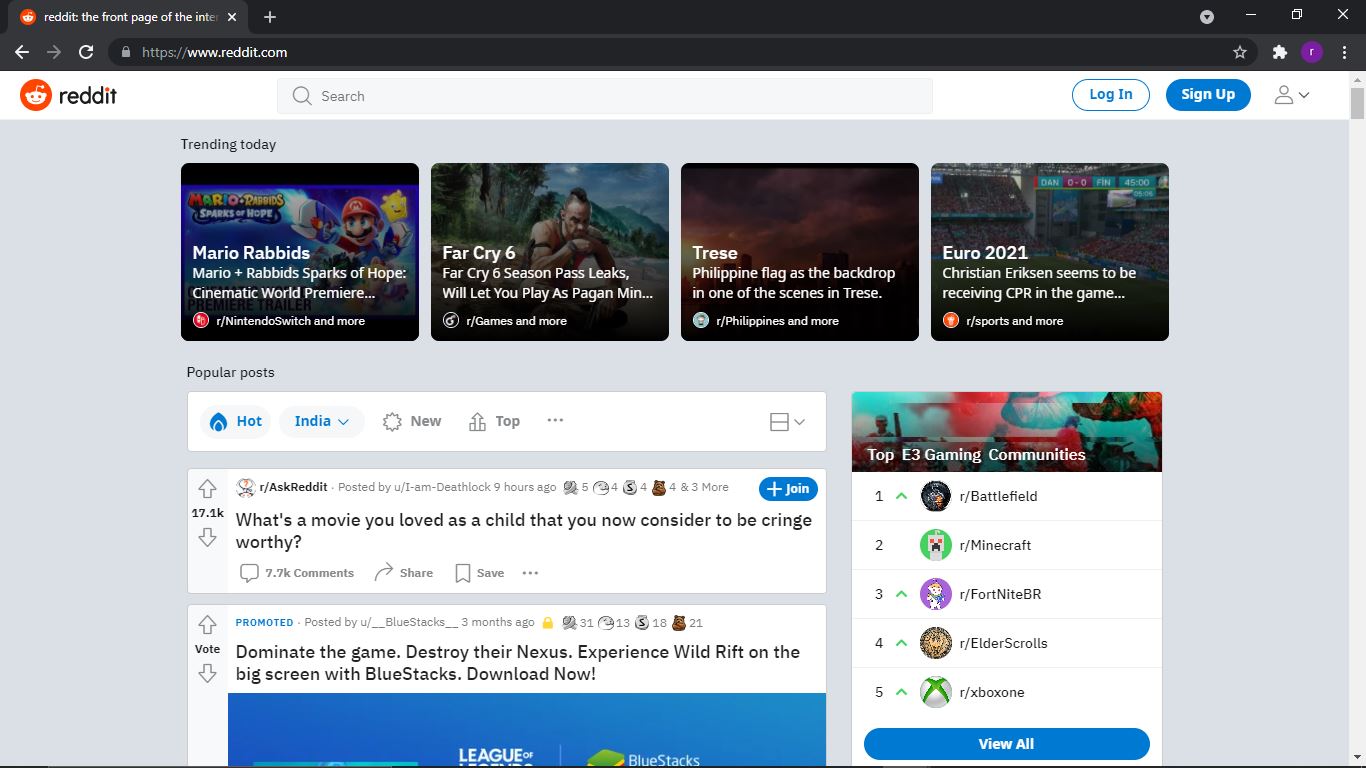**Screenshot of Reddit's Interface: Detailed Description**

At the very top of the image, we see a browser tab title which reads "Reddit, the front page of the..." with the remainder of the title truncated. Next to this title is the standard 'X' button for closing the tab. Notably, no additional tabs are open. Below the tab title, the browser's navigation bar is visible with back and forward arrows (the forward arrow is grayed out), a refresh icon, and a security padlock icon indicating a secure connection. The URL displayed is "https://www.reddit.com."

Directly beneath this, the Reddit header is situated, featuring the Reddit logo followed by the word "Reddit." There's a search bar available for users to input queries, with "log in" and "sign up" options to the right. The "log in" button is presented in white text on a blue background, while the "sign up" button reverses these colors. Additional profile management options are available through a small profile icon with a downward arrow.

Below the header, a "Trending Today" section is prominently displayed, featuring four small images with accompanying labels:
1. **Mario Rapids** - An image of Mario.
2. **Far Cry 6** - A depiction of a warrior standing on a beach.
3. **Trese** - Possibly spelled T-R-E-S-E, accompanied by imagery of a dark sky.
4. **Euro 2021** - A distant view of stadium stands.

Under the trending section, the interface proceeds to the "Popular Posts" area, seemingly filtered by 'hot' and then 'India'. The first visible post is from the subreddit **AskReddit** with the title, "What's a movie you loved as a child that you now consider to be cringeworthy?"

Embedded within this list of posts is a promoted advertisement reading: "Dominate the game, destroy their nexus, experience Wild Rift on the big screen with BlueStacks. Download Now."

On the far right side of the page, there's a sub-menu titled "Top E3 Gaming Communities," which lists five notable gaming communities without specifying further details in the text.

This detailed description encompasses all the elements visible in the provided screenshot of Reddit, offering comprehensive insights into the webpage layout and content.